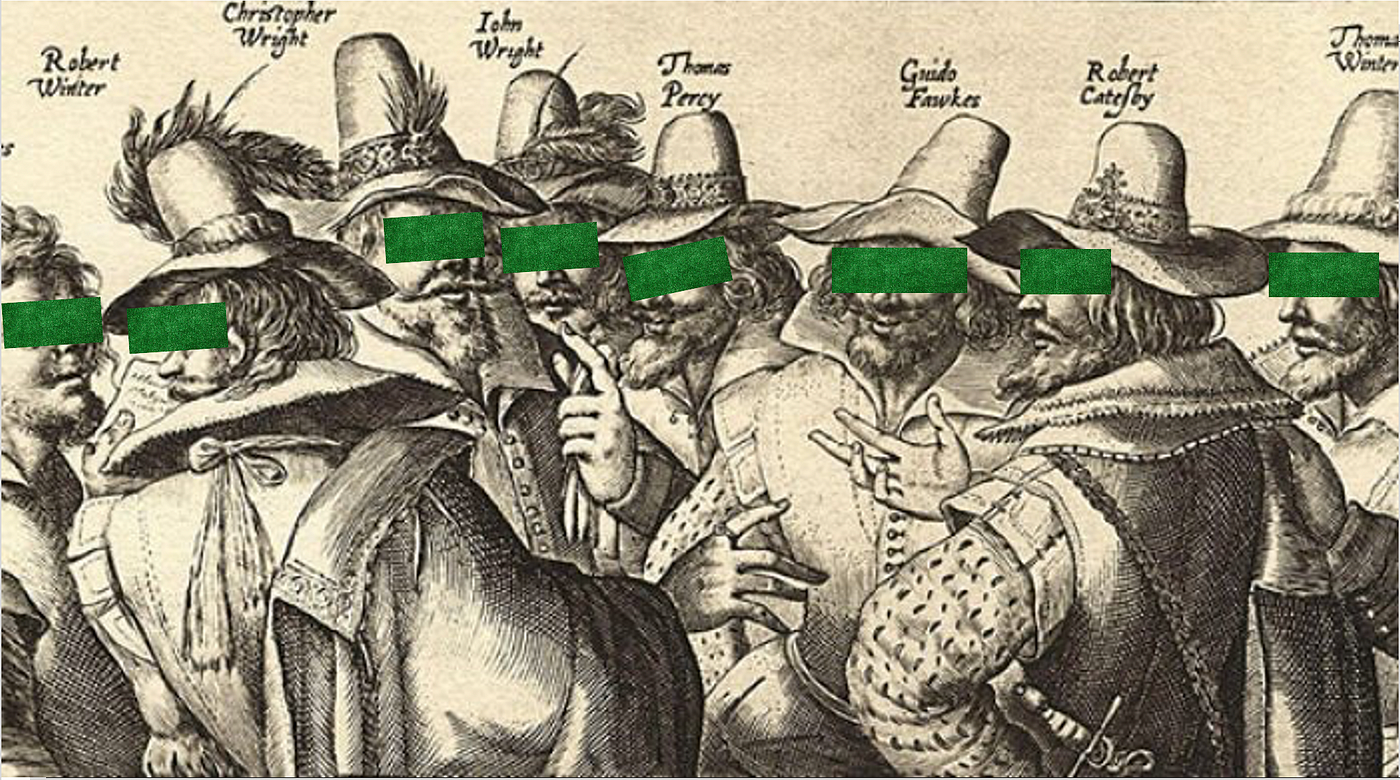This rectangular black and white pencil sketch, approximately six inches wide by three inches high, is drawn on light brown parchment. It depicts eight men from the waist up, all in period clothing with long hair, beards, and mustaches. They each wear conical hats with floppy brims adorned with feathers and are dressed in shirts with short sleeves and have purses slung over their shoulders. Their long, skinny fingers stand out against their vintage attire. Above each man, their names are inscribed in bold black print: from left to right, they are Robert Winter, Christopher Wright, John Wright, Thomas Perry, Guido Fox, Robert Cadeffy, and Thomas Winter. A distinctive feature is the small green rectangle obscuring each man's eyes, adding a modern, mysterious touch to the historical portrayal.